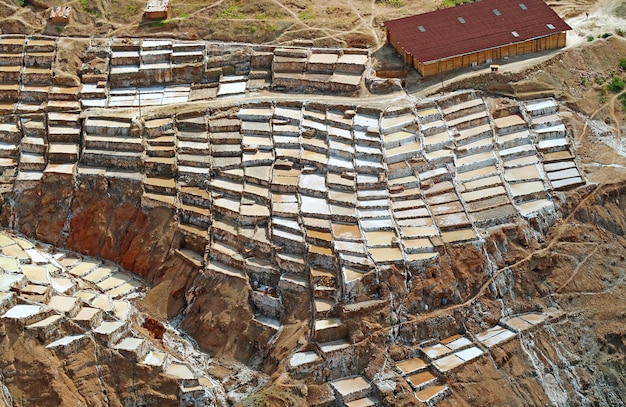The image features an aerial view of a sunlit quarry or mining operation, characterized by a uniquely terraced, rocky landscape. The terrain appears as slabs of stone fractured and cut into square and rectangular shapes, creating a grid-like pattern reminiscent of rice paddies but composed of various shades of granite and rock. The scene showcases these multicolored slabs—ranging from rust, tan, black, white, gray, and multiple shades of brown—stacked in rows and columns. In the background, patches of grass can be seen, providing a natural contrast to the industrial activity. Dominating the upper right corner is a flat, light brown warehouse-like building with a reddish-brown roof featuring several sunlit windows. This setting combines natural geological formations with human mining efforts, resulting in an intriguing, geometrically shaped landscape.